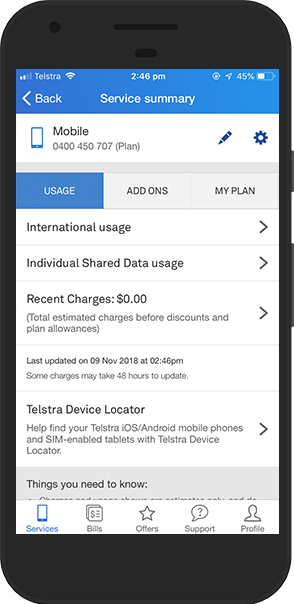This image depicts an iPhone screen with the Telstra carrier network displaying at the top. The battery level is at 45%, and the current time is 2:46 p.m. The signal strength indicator shows a very strong connection. 

The interface features a navigation menu with a left arrow labeled "Back" and the heading "Service Summary." Below this, there are several sections highlighted including:

- **Mobile:** Accompanied by an icon of a mobile phone.
- **Usage:** This is highlighted in blue, with associated sections like "Add-ons" and "My Plan" displayed in gray.
- **International Usage:** Indicated by a right-pointing arrow.
- **Individual Shared Data Usage:** Also indicated by a right-pointing arrow.
- **Recent Charges:** Currently shows a value of zero and includes a right-pointing arrow.
  
The screen notes the last update as occurring on November 9th, 2018, with a timestamp provided. There is a mention of the "Telstra Device Locator," which includes a right arrow and a brief description stating it helps locate Telstra iOS, Android mobile phones, and SIM-enabled tablets.

Near the bottom of the screen, a message begins with "Things you should know," but this content is cut off in the image. There are also icons at the bottom for navigation, which include: 

- **Services**
- **Bills**
- **Offers**
- **Support**
- **Profile**

These icons suggest various functionalities available to the user within the app.